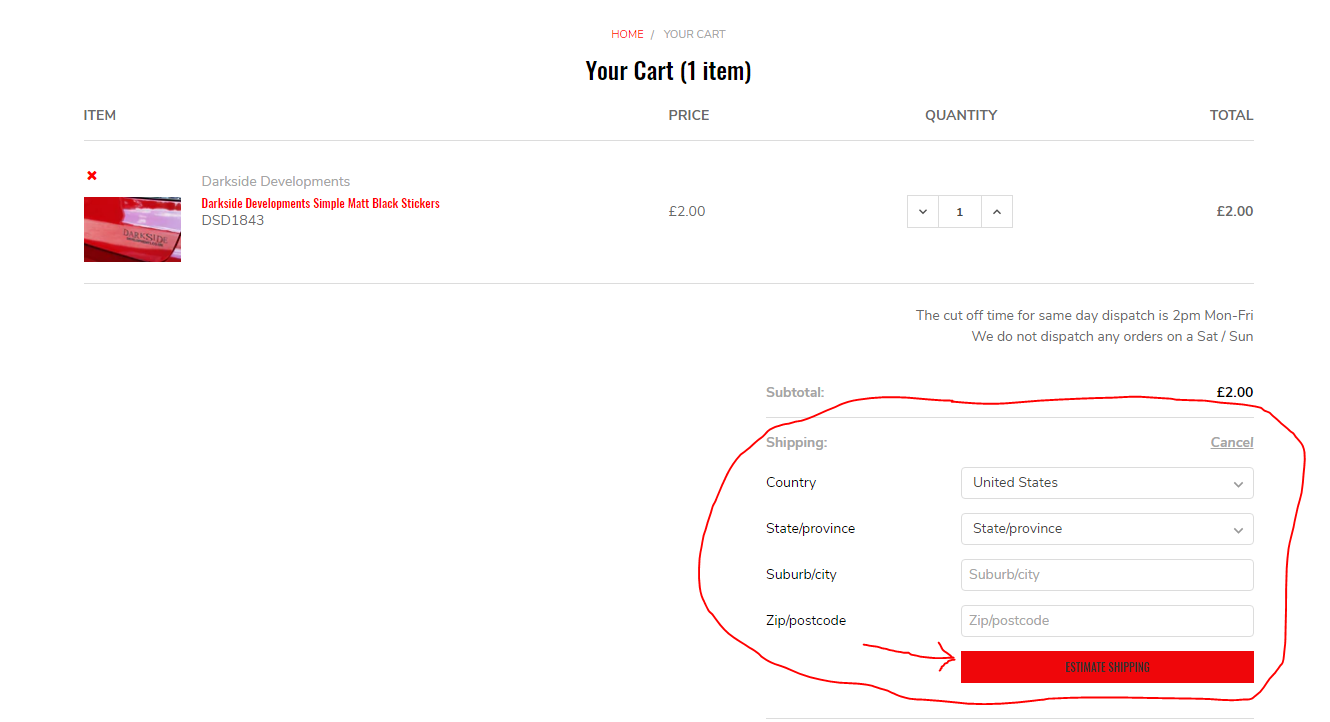This image showcases a blurred and pixelated screenshot of a webpage with a white background, displaying less than optimal quality and resolution. The top and middle parts of the webpage are labeled "home.com" and "your cart.com" respectively. Below this header, there are four distinct columns labeled "Item," "Price," "Quantity," and "Total."

Under the "Item" column, there's an indistinct red image, its details obscured due to the low resolution. To its right, readable text says "Dark Side Developments," beneath which there is another block of illegible red text. In the "Price" column, the value displayed is "2€" (or 2 pounds), and the "Quantity" is marked as "1." Correspondingly, the "Total" column lists the amount "2€."